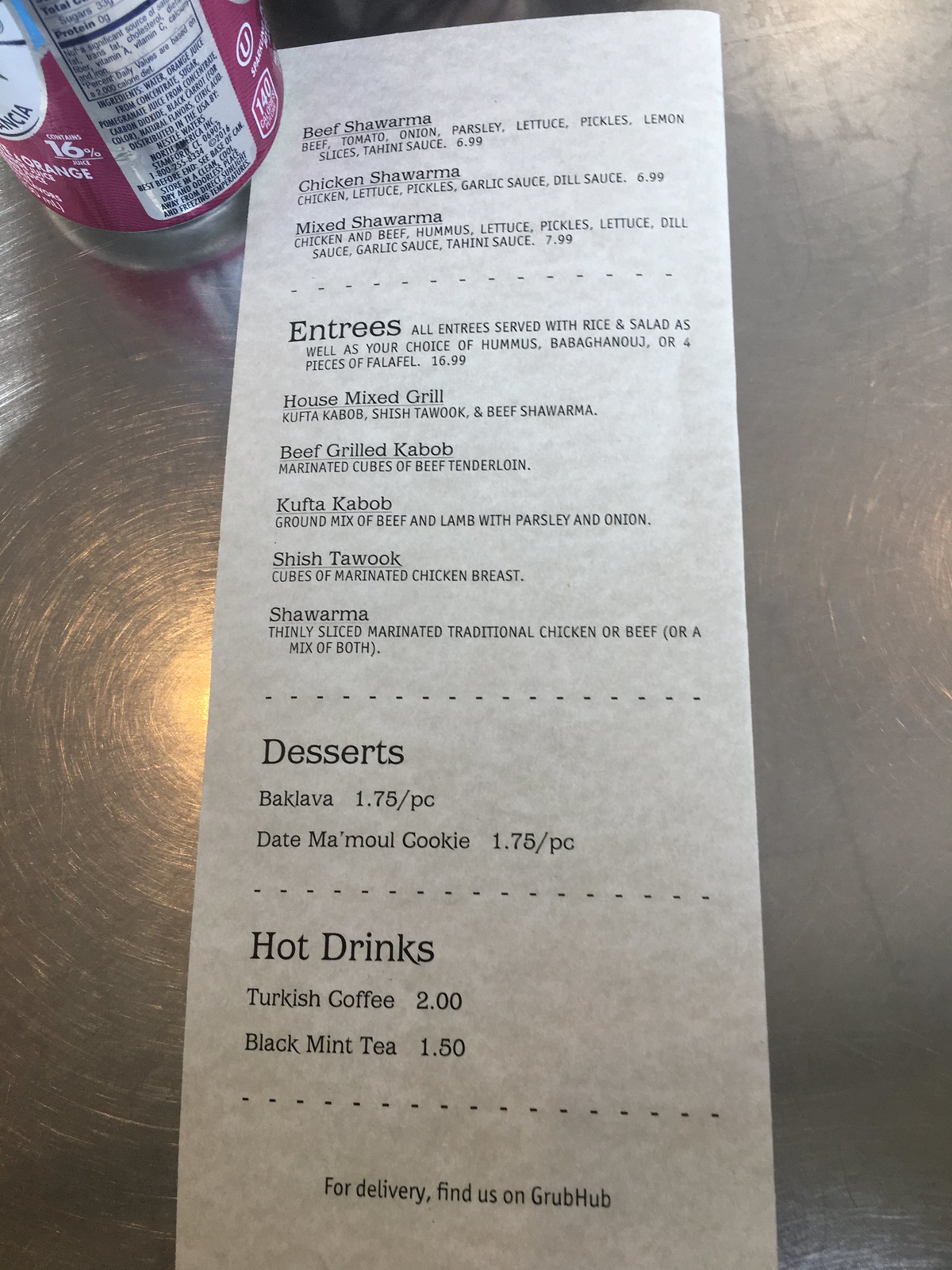This color photograph, taken in portrait mode, showcases a vertically positioned, narrow menu printed on white parchment-style paper. The menu starts with a list of three appetizer selections at the top: Beef Shawarma, Chicken Shawarma, and Mixed Shawarma. Below this section is a dotted line, followed by a detailed entrée list featuring: House Mixed Grill, Beef Grilled Kebab, Kofta Kebab, Shish Tawook, and Shawarma. Beneath another dotted line, the dessert options are displayed, which include Baklava and Date Mamoul Cookie. The final section, separated by yet another dotted line, highlights the available hot drinks: Turkish Coffee and Black Mint Tea. An additional dotted line at the bottom provides a call-to-action for delivery, suggesting customers find the establishment on Grubhub.

The menu is set against a reflective, shiny metal table, with light softly glinting off its surface from above. In the upper left corner of the image, a dark red beverage can with a silver nutritional label and some white text partially overlaps the top edge of the menu. The specific type of drink is not discernible due to the angle of the can.